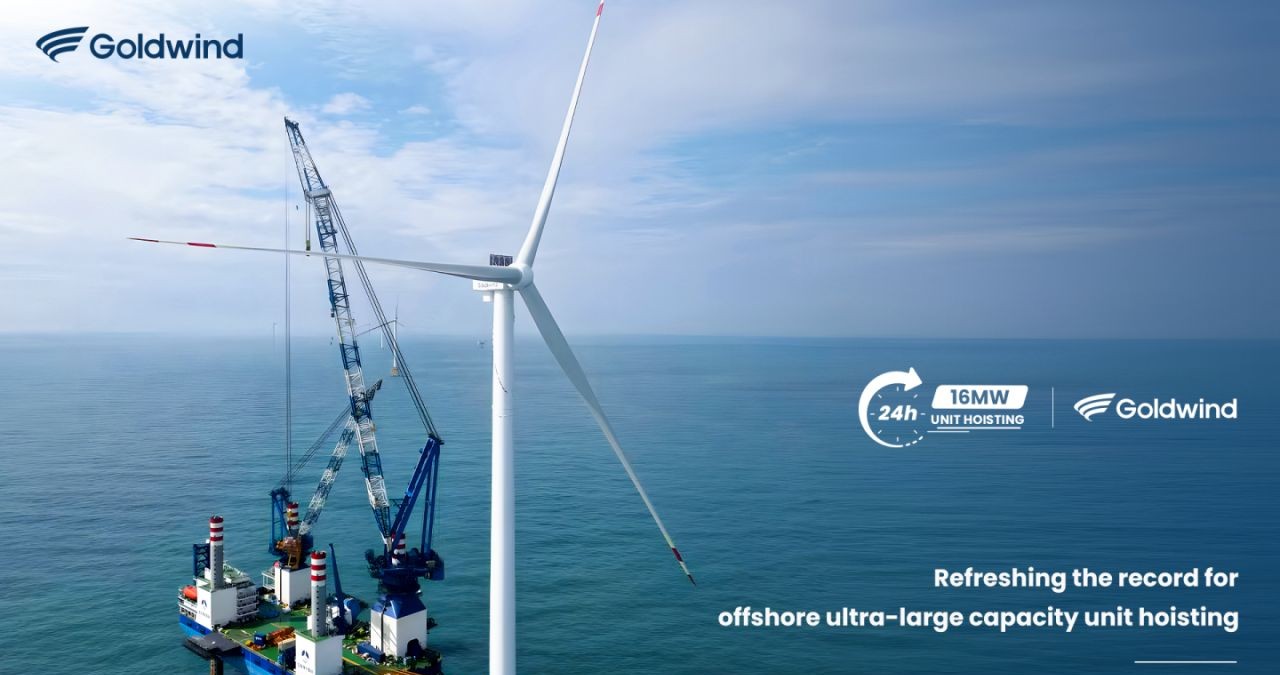The image is an advertisement for Clean Energy from Gold Wind, featuring a striking scene of the ocean under a vast blue sky with scattered clouds. Dominating the left side of the image is a towering white wind turbine on a platform, symbolizing offshore renewable energy efforts. The top left of the image includes the logo "Gold Wind," while the bottom right displays the text: "Refreshing the Record for Offshore Ultra-Large Capacity Unit Hoisting." A high-angle view reveals the platform—a green, rectangular structure with blue buoys extending into the water, white towers on each corner, and a blue and white crane prominently positioned. Ironically juxtaposed in the background is an offshore oil platform, adding an element of contrast with its tall white towers capped with red and white stripes. The scene underlines a transition towards sustainable energy while maintaining traditional imagery.